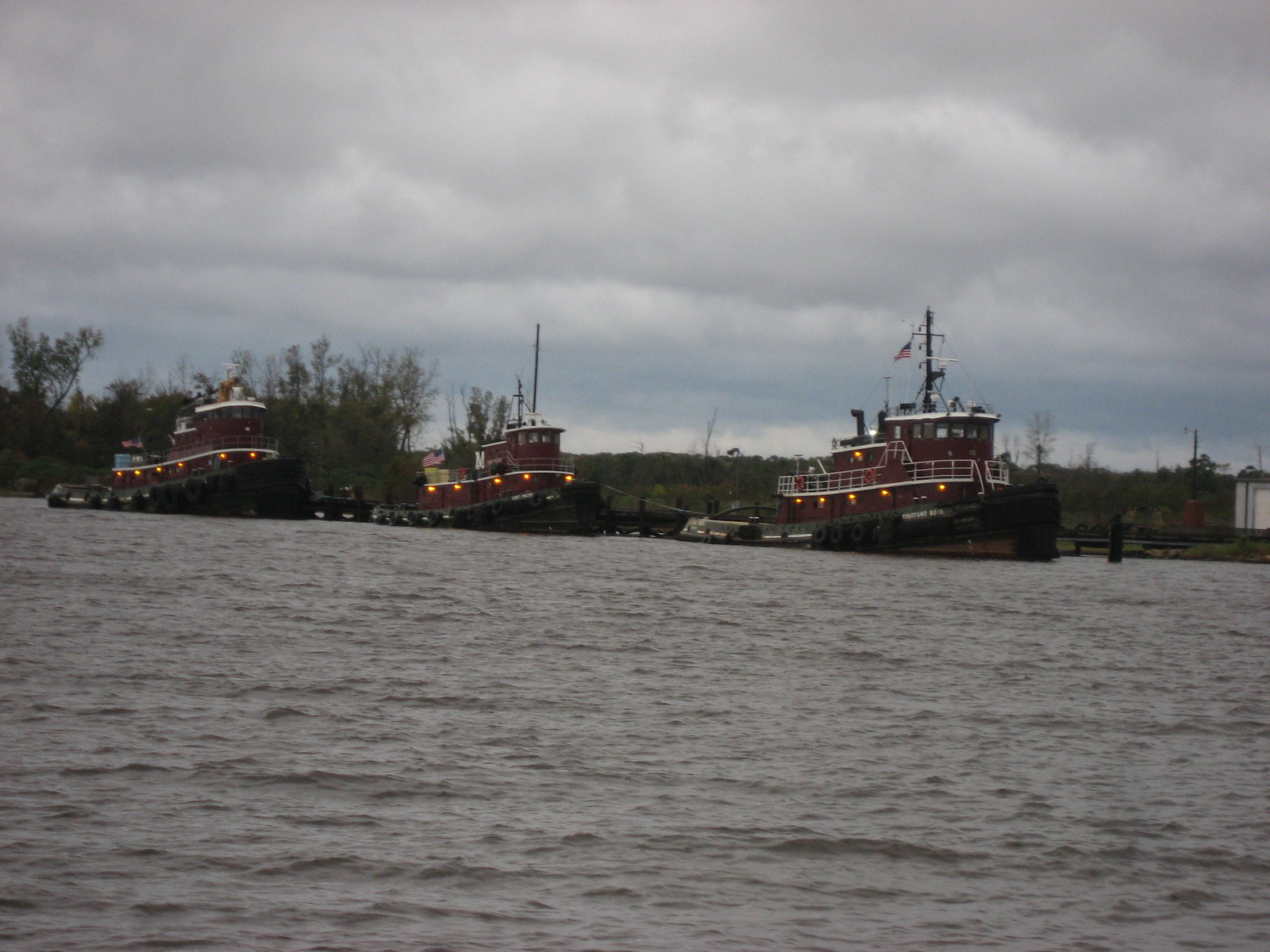This photograph captures a dreary, cloudy day at a gray, slightly wavy body of water occupying the lower half of the frame. Three stationary tugboats, each about 30-35 feet long, float near the shore. These tugboats share a consistent color scheme with black hulls and red upper structures, and each is adorned with an American flag. The leftmost tugboat features a prominent mast, while the tugboat in the middle displays what looks like the letter "M." The rightmost tugboat is equipped with two red life preservers on its railing. In the background, bare trees and a small shed-like building are visible under the overcast sky, suggesting a cold, northeastern climate.